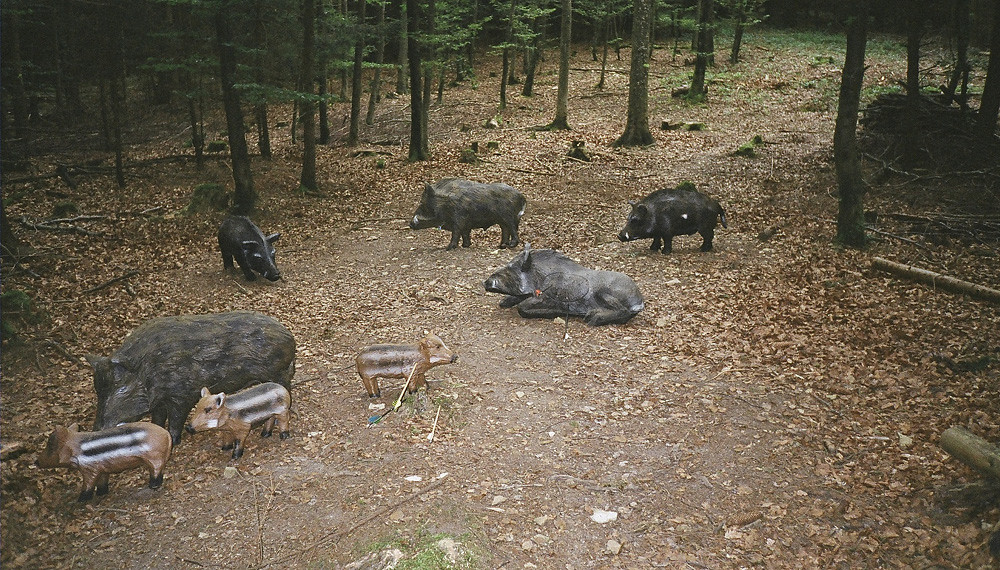In this detailed color photograph taken in landscape mode, we see eight animal statues positioned in a forest setting on a dirt-covered area scattered with brown and yellow leaves. The foreground features three smaller statues resembling large rodents, possibly young capybaras, with distinct black and white stripes running horizontally across their brown bodies from their shoulders to their rear. These smaller statues align near the largest adult statue in the lower right corner. Surrounding them are five larger statues, three to five times the size of the smaller ones, resembling boars or warthogs with sturdy bodies, tapered snouts, and small white curved tusks. One of the larger statues lying in the center faces left, while the others stand or mill around. One notable larger statue has a white stripe that extends over its nose, across its head, and onto its back. The background is filled with trees with green leaves, creating a shadowy, canopied forest atmosphere that gradually fades into darker green hues, indicating dense foliage and an overcast day.